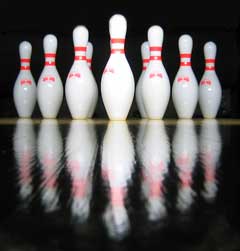A color photograph captures a pristine setup of ten traditional white bowling pins, each featuring two bold red stripes around the neck and a faint red insignia below. The pins are arranged in the classic triangular formation, ready for a perfect strike. The setting against a stark black background enhances their prominence, while their clear reflections ripple across a glossy black surface at the base. A thin yellow line subtly bisects the image just below the pins, adding a touch of contrast. The scene is devoid of any people, animals, plants, buildings, or vehicles, focusing solely on the pristine, reflective arrangement of the bowling pins.